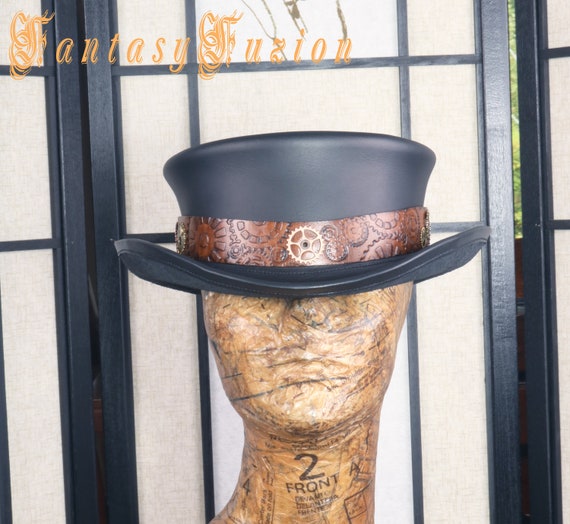The photograph features a close-up view of a mannequin head and neck, positioned against a glossy black lacquered folding partition with white rice paper panels, reminiscent of an Asian room divider. The mannequin itself has a rough, cork-like texture, suggesting a material akin to paper mache or wood. It displays a weathered look, with details of a face, including the nose and mouth, slightly discernible. Notably, the neck of the mannequin bears vintage map-like prints and markings, including a number two and the word "front."

The centerpiece of this image is the hat adorning the mannequin. The hat resembles a short top hat, combining elements of both bowler and police hat styles, with a brim that extends uniformly around. Encircling the hat is a distinctive band, styled like a tooled leather belt, adorned with intricate steampunk gears and clock mechanisms. 

Adding a touch of fantasy, a watermark of stylized orange text overlays the top left corner of the photograph, reading "Fantasy Fuzion" in an ornate medieval font.